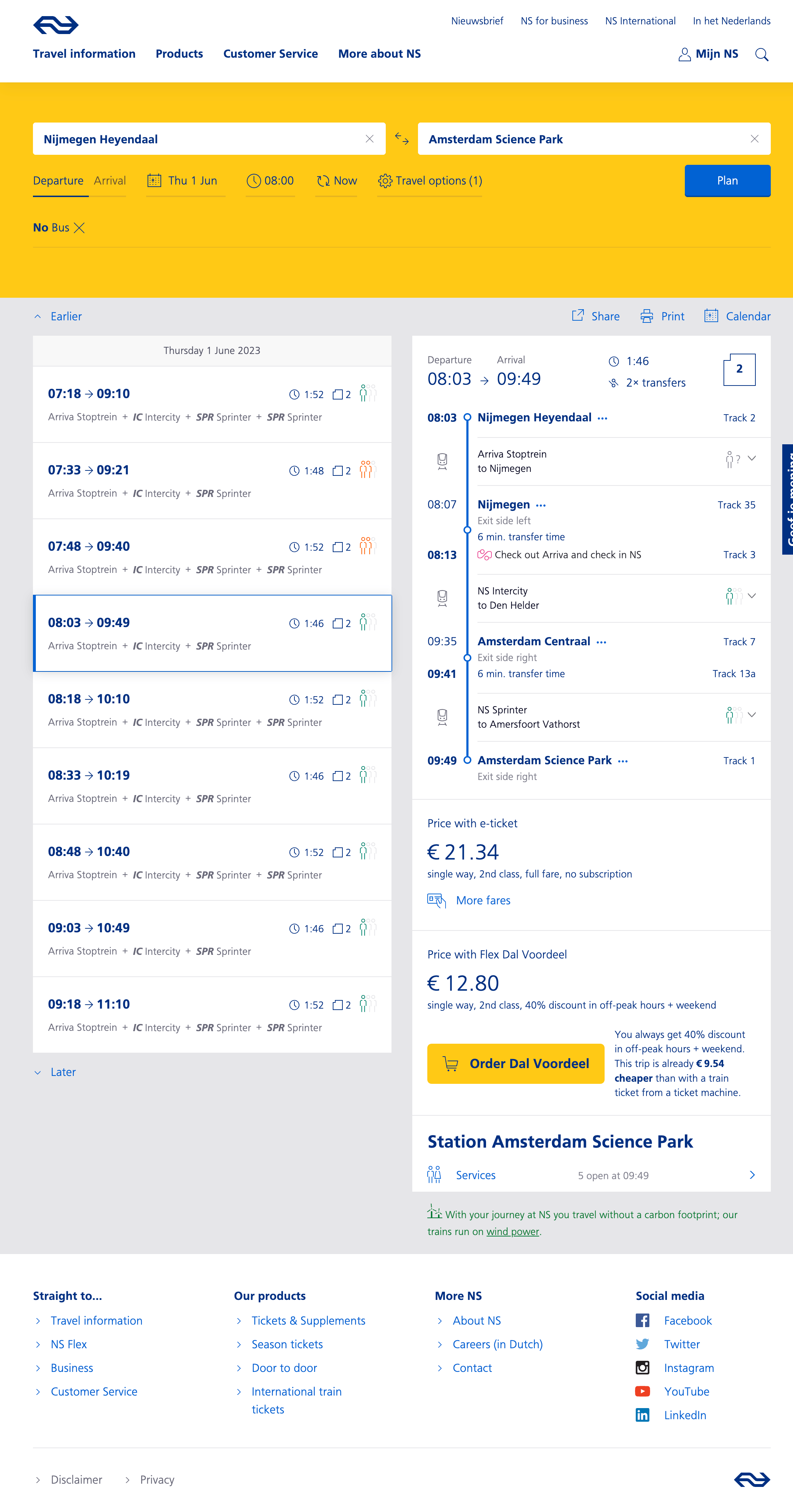This image displays a detailed layout of a website. In the top left corner, the site features various categories such as "Information," "Products," "Customer Service," and "More About the Company." The company logo is distinct, resembling a swirling symbol.

Dominating the center of the webpage is a large gold box, within which are two smaller white input boxes likely meant for user information. Adjacent to this, a blue clickable box is present, although the white text inside it is too small to discern clearly.

The website is divided into two main sections. Both sections feature lists accompanied by numbers with gray headers at the top, which also contain unreadable text. Along the left side of these sections, there are purple digits followed by additional text, while similar digits and writing appear on the right side.

Several icons are scattered across the page, including two red trash icons and various blue icons on the right side of some items. A vertical dividing line separates the sections, denoting different types of content.

Toward the bottom, there is additional information with the numbers 2134 and 1280 appearing near phrases like "order chat"—although the exact wording is unclear due to its small size. Finally, the footer of the webpage prominently displays "Station Amsterdam Science Park."